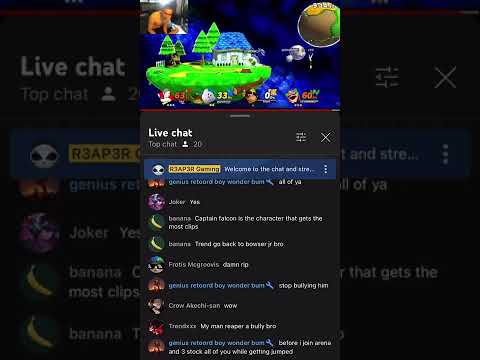This image is a complex screenshot of a live chat that layers another screenshot within it. The primary screenshot displays a live chat interface, but embedded within it is another screenshot where the background chat is blacked out. 

In the embedded screenshot, there is a detailed illustration featuring a picturesque village set against a lush, green landscape complete with pine trees. A specific house stands out, painted with a blue roof and enclosed by a small fence. Departing from this tranquil village scene is a spaceship heading towards Earth, adding a twist of sci-fi to the idyllic setting. Positioned below the village are various characters likely created by the chat's organizer, serving as inhabitants of this fictional place.

The text overlay on the live chat is quite vivid, capturing conversations between participants with usernames such as Genius, Reford Boy, Wonder Trait, and Joker. Highlights include multiple clips, mentions of characters like Captain Falcon and Brodus MacGullivis, and chaotic dialogue reflective of an active and engaged community. Notable statements include Genius' plea against bullying, Cro-A-Hachi-San's expression of astonishment, and Transdex's commendation of "Reaper." The conversation culminates in Genius' assertion about joining and stacking against multiple participants, hinting at a highly competitive or playful interaction amongst the users.